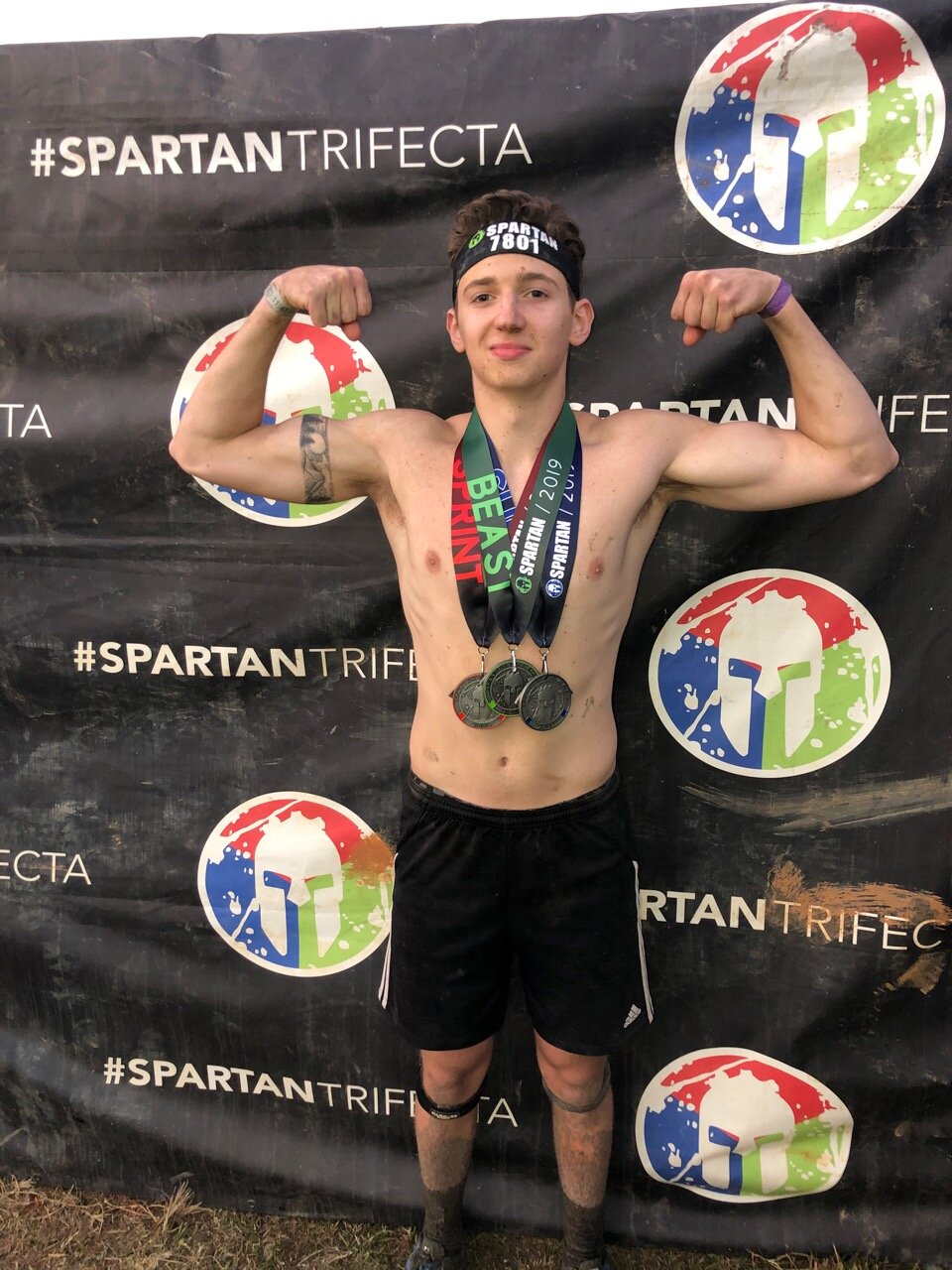A young man, likely in his late teens or early 20s, proudly poses in front of a mud-splattered event backdrop with the hashtag "Spartan Trifecta" and a Spartan mask symbol featuring red, green, and blue triangles within a white circle. Shirtless and flexing his biceps, he wears black athletic shorts, a Spartan 7801 headband, and three medals with "Spartan 2019" inscribed on them—each adorned with a distinct ribbon in green, red, and blue. His brown hair is spiked up, and his brown eyes shine with pride. He has a tattoo around his right bicep and sports two Livestrong-style bracelets, one on each wrist. This image captures his sense of accomplishment and the triumphant end of a challenging race.